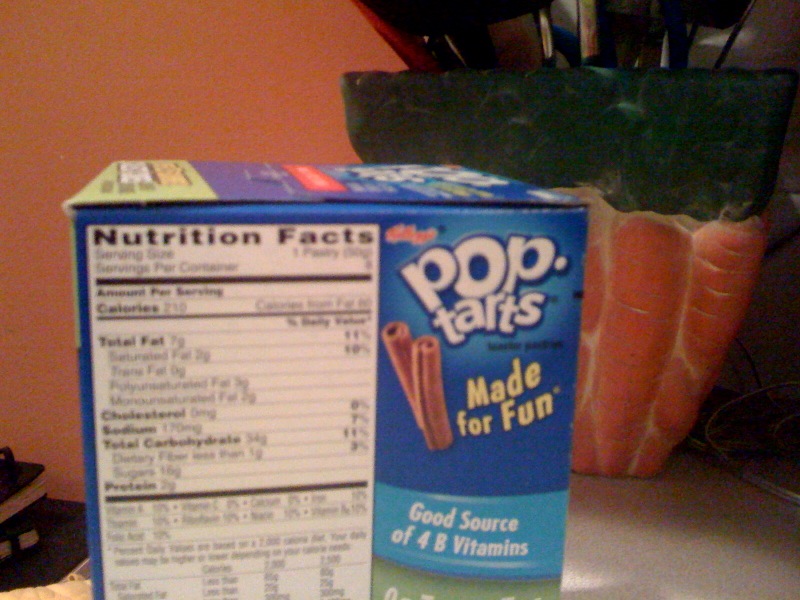The image captures a box of Pop-Tarts displayed prominently on a table. The box is the standard blue packaging commonly associated with Pop-Tarts, though it does not indicate the specific flavor. On the right side of the box, the iconic "Kellogg's Pop-Tarts" logo is clearly visible. To the left, the nutritional facts are presented in black lettering on a white rectangular background, starting with the calorie count and continuing downward. Despite some blur, the bold "Nutrition Facts" header remains readable. Additionally, a swinging banner at the bottom of the box highlights that it is a good source of 4 B vitamins.

The box sits on a plain table, and in the background, there is a pot, presumably containing a plant. The setting appears to be indoors, although only a portion of the room is visible. The backdrop seems to be an orange-hued wall, providing a warm tone to the overall composition.